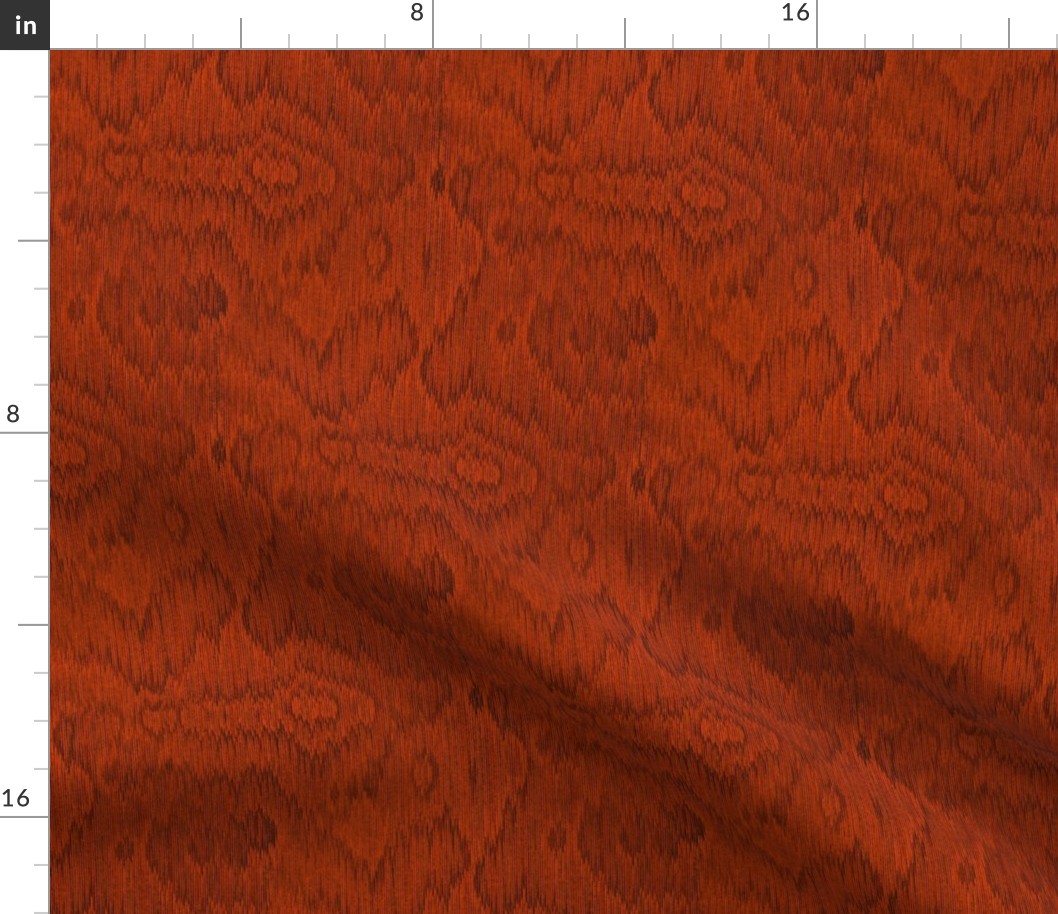The image depicts a detailed, scaled illustration with a textured surface that appears to be red or orange. At the top left corner, there's a small black square containing the letters "IN" in white, which likely indicates inches. Surrounding the central textured area is a measurement gauge, with notches and lines that repeat along the top and left sides. The gauge includes larger lines marked with the numbers 8 and 16. The texture within the image seems reminiscent of wood grain or fabric thread, featuring darker lines resembling wrinkles or swirls that enhance the intricate design.